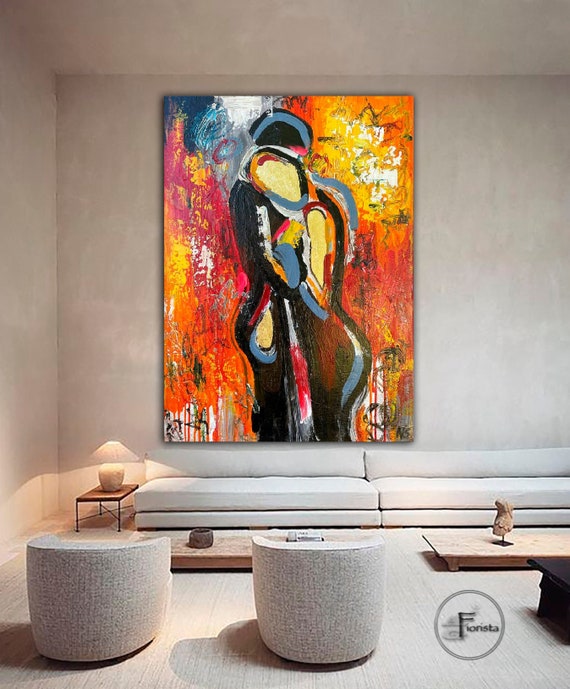The image depicts a high-ceilinged living room with a minimalist, high-end design theme dominated by white and cream colors. The focal point of the room is a large, vibrant abstract painting mounted on a light brown wall. The painting portrays two people, a man, and a woman, embracing, with bright colors such as orange, red, yellow, blue, black, and touches of magenta and white. Below this striking piece of art, there is a long, low-lying beige or cream sofa without visible legs. To the left of the sofa stands a small, lit lamp with an angular shade, placed on a small wooden end table. Facing the painting, there are two round, white chairs and two very low wooden coffee tables, one of which holds a decorative sculpture. The room's understated elegance is punctuated by the colorful painting, creating a striking contrast. Additionally, the bottom right of the image features a circular logo with the word "Fiorista," suggesting this might be an advertisement for a design studio.